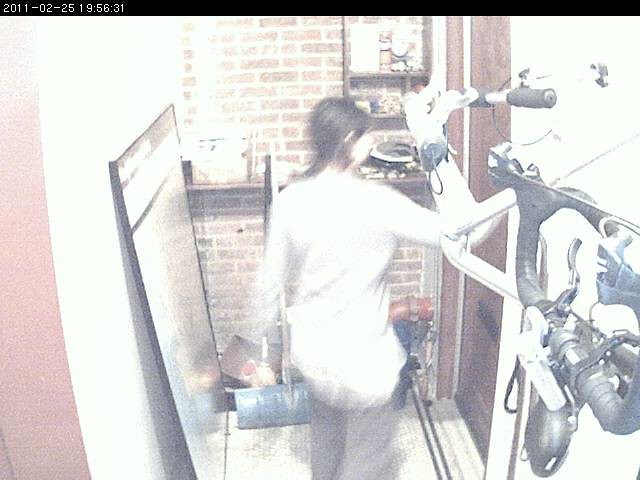This image appears to be an overexposed and pixelated color photograph, creating a faded effect that compromises visibility and blurs many objects. At the very top of the image, a thin black band runs across the rim, displaying a series of numbers, potentially indicating a date and time: 2011-02-25-1958-31. Dominating the center, we see the back of a woman with longish hair, slightly turned towards the right. She is dressed in a long-sleeved white or light gray shirt and possibly light gray trousers. She seems to be standing or perhaps leaning slightly, possibly in an indoor space that resembles a gym or a hallway.

Behind her is a distinctive brown and white brick wall, with a white wall to the left. A large rectangular reflective object, possibly a mirror or a framed picture, is propped against this white wall. To the very far left, a pale reddish wall suggests that we might be peering into the room through a doorway. Additional details include instruments atop a shelf, and to her right, gray or silver equipment that could be gym apparatus or pipes, further lending to the gymnasium-like atmosphere. A notable feature on the right wall is a brown door with a mail slot at the bottom. The overall scene is difficult to discern with precision due to the photograph's faded, grainy quality, and overexposed lighting.